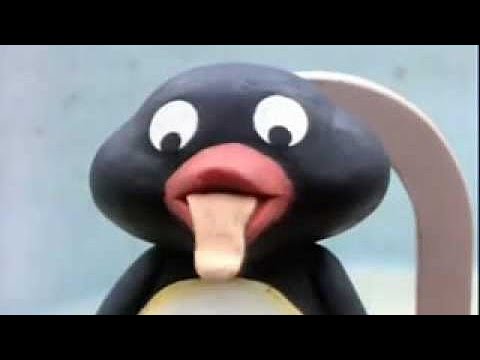This 3D-rendered cartoon character, reminiscent of claymation, sits in a white, arched-back chair against a bright, baby blue background. Framed by black stripes at the top and bottom (and a tiny black border on the right side), the character is predominantly black. It features a black, oval-like head and body, with a distinct white round shape at the center of its torso. The character's large, round white eyes with black pupils gaze downward. It has a reddish-pink beak with a light orange or yellow tongue sticking out. The overall design suggests a penguin-like creature with a distinctly whimsical and playful appearance.